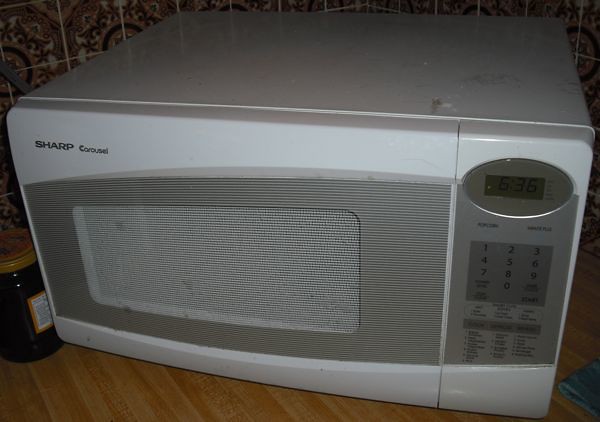This is a detailed photograph of a white Sharp Carousel microwave with a gray front panel, positioned centrally on a brown wood countertop. The brand name, "Sharp Carousel," is visibly marked on the top left of the microwave's facade. The digital display and number pad are situated on the right-hand side, both in varying tones of gray. The microwave, presumed to be an older model, appears powered off, with its black digital display inactive.

In the foreground, to the left of the microwave, is a jar of jam or jelly, adding an element of daily use to the scene. The countertop is nestled into a corner, and the microwave seems slightly pushed into this space. A small piece of cloth peeks out from the front right corner of the microwave. The backdrop features a decorative red and white patterned wall, blending seamlessly with a circular design motif that adds an artistic touch to the setting. The overall image is slightly low-angled, capturing both the top and front views of the microwave. There is noticeable dirt on both the top and the front of the appliance, indicating frequent usage.